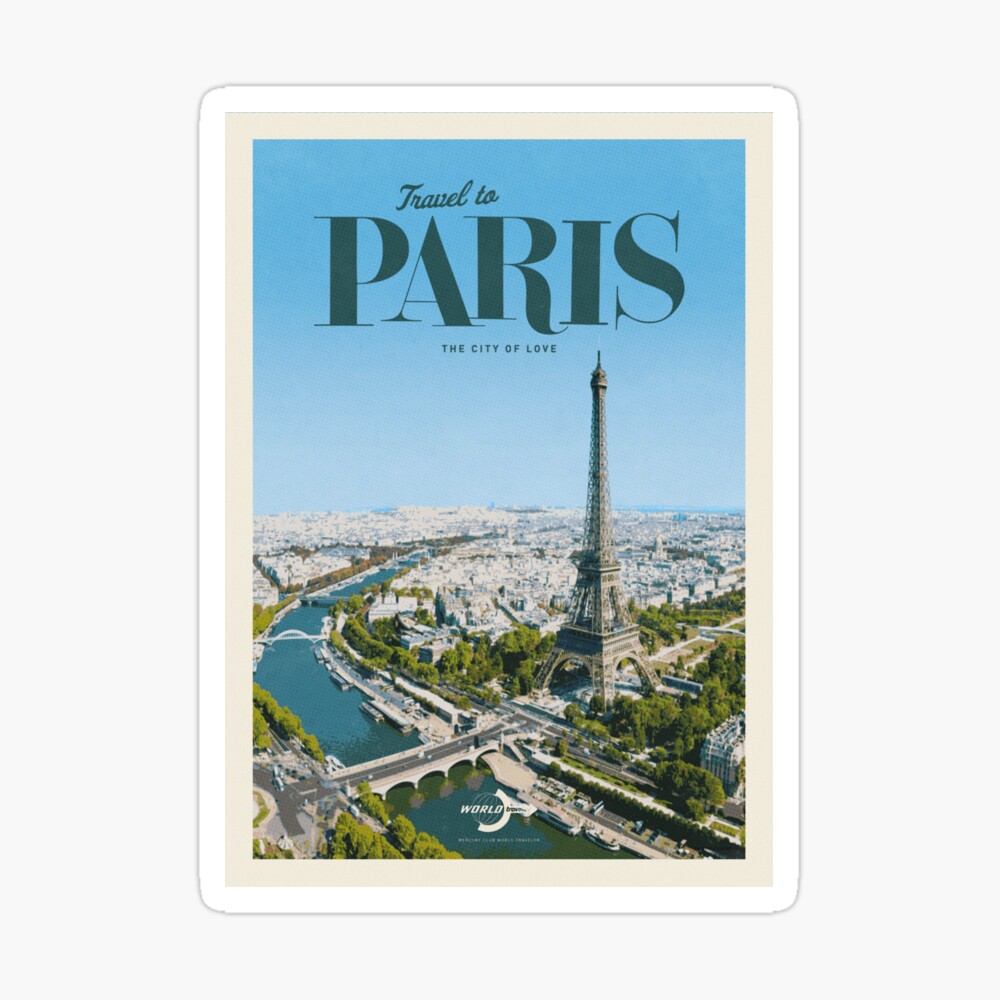The image captures a highly detailed and visually captivating aerial view of the Eiffel Tower in Paris, surrounded by an intricate network of streets, buildings, bridges, and the river Seine. The scene is framed by a white border that encloses a light pink trim, lending it a postcard or advertisement feel. The elegant composition highlights the lush greenery and tree-lined paths, especially notable from the trees curving around the Eiffel Tower and extending towards the left. Dominating the top of the image is a clear, gradient sky shifting from a dark blue at the uppermost point to a lighter blue where it meets the cityscape. The atmosphere is enhanced by a bridge extending from the Eiffel Tower to the bottom left, underlining the city's intricate beauty.

At the top of the image, the text "Travel to Paris" is elegantly written in black, with "Paris" in larger and bolder font, three to four times the size of the accompanying text, and beneath it, in much smaller letters, is the phrase "the city of love." The bottom of the image bears a globe icon featuring the word "world" within it, trimmed halfway in white. The captivating details and vibrant, bright colors along with the clear emphasis on architectural beauty and natural elements make the city appear as an enticing and romantic destination, ideal for tourists.